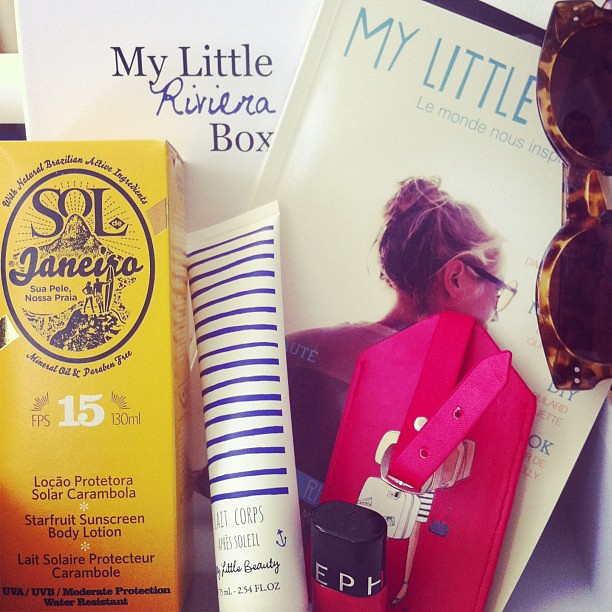This image features a stack of books with intriguing items placed among them. At the top of the stack, a pair of tortoise shell sunglasses with dark lenses rests, partially covering a book. The title of this book, in blue lettering, reads "My Little" followed by the obscured text "Le Monde Nou..." and "INSU...", with an image of a woman on the cover who has her hair up in a bun and appears to be wearing glasses. Over this book is a pink luggage tag, adding to the eclectic mix of items. Beside the book is another titled "My Little Riviera Box," which lies below a small wallet-like item and a tube of white cream with blue stripes, potentially hand lotion, labeled with details such as "Cor Apa Soleil, Little Beauty, 2.54 fluid ounces." Additionally, there is a box labeled "SOL 15," likely containing suntan or sunscreen, and adjacent to this is a pink nail polish bottle. The yellow container with brown lettering, possibly another sunscreen product, adds to the scene, making for a visually engaging and detailed composition reflecting a collection of travel and beauty essentials.